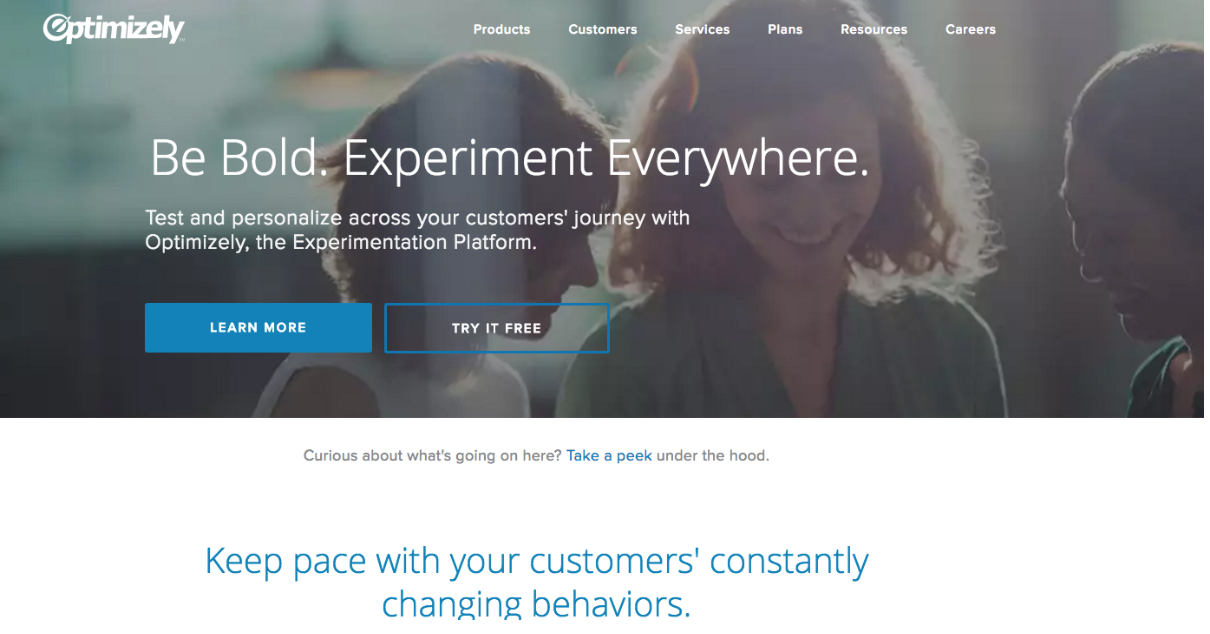This is a detailed caption of an image depicting a website's landing page:

The screenshot captures the top half of the website's landing page, featuring a visually engaging background image. The background shows three women standing close together, all gazing down at an object that is not visible in the frame. One woman, situated slightly to the right of the center, faces the camera while looking down. The other two women, positioned on either side of her, are in profile, also looking down.

At the top left corner of this background image, the Optimizely logo is prominently displayed in white text. To the right of the logo, there is a horizontal menu bar with six categories, all written in white sans-serif text. They are, from left to right: Products, Customers, Services, Plans, Resources, and Careers.

Centrally placed within the background image, yet slightly off-center to the left, is the headline text in large white font: "Be Bold, Experiment Everywhere." Directly below this headline, a smaller white text reads: "Test and Personalize Across Your Customer's Journey with Optimizely, the experimentation platform."

Further down, two call-to-action buttons are displayed. The first button, in solid blue with white text, says "Learn More." Next to it, a blue translucent outlined button reads "Try It Free."

Below the background image, the page transitions into a section filled with white negative space. A small line of text in gray reads: "Curious About What's Going On Here? Take a Peek Under the Hood," with "Take a Peek" highlighted in blue. Finally, large blue text declares: "Keep Pace With Your Customer's Constantly Changing Behaviors," though the bottom parts of the Gs in "Changing" are cut off by the bottom edge of the screenshot.